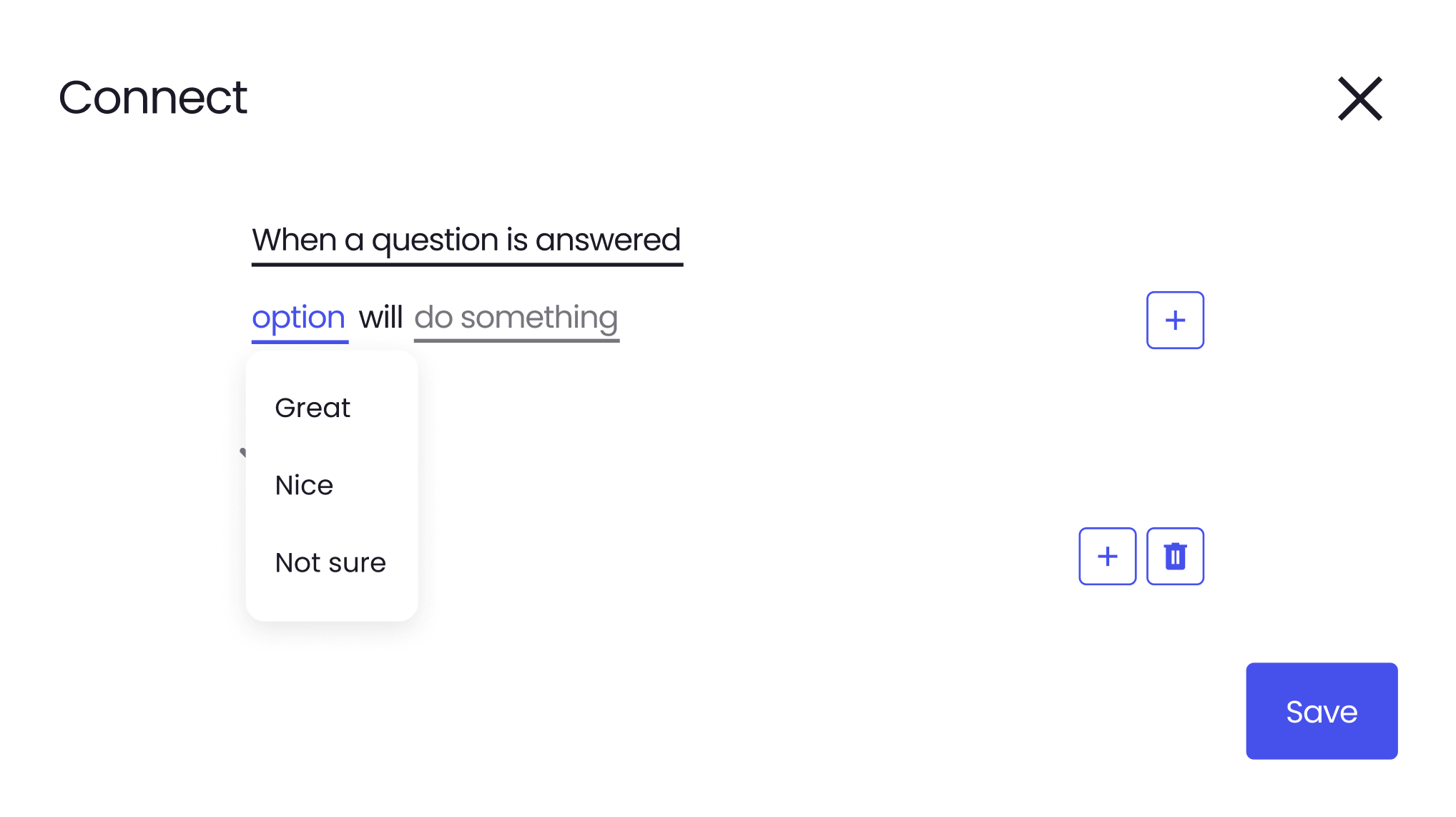This image depicts a user interface of an auto-correct program set against a white background. At the top, there is a header featuring the black text "Connect," flanked by a large, slightly blurry black "X" on the right. Directly below, a sentence is underlined: "When a question is answered, option will do something." In this sentence, the word "option" is highlighted in blue, while "do something" appears in dark gray. Under "option," a drop-down menu presents several choices in black text against a white background. The options available are "Great," "Nice," and "Not sure." 

To the right of the drop-down menu is a blue plus sign inside a blue box. Below this, there are two smaller blue icons: a plus sign within an outlined blue square and a trash can symbol inside another outlined blue square. Finally, situated in the bottom right corner is a larger, filled, bluish-purple rectangular button with white text that reads "Save." Overall, the photo captures a functional yet slightly blurred aspect of the interface, focusing on elements crucial for user interaction within the auto-correct program.